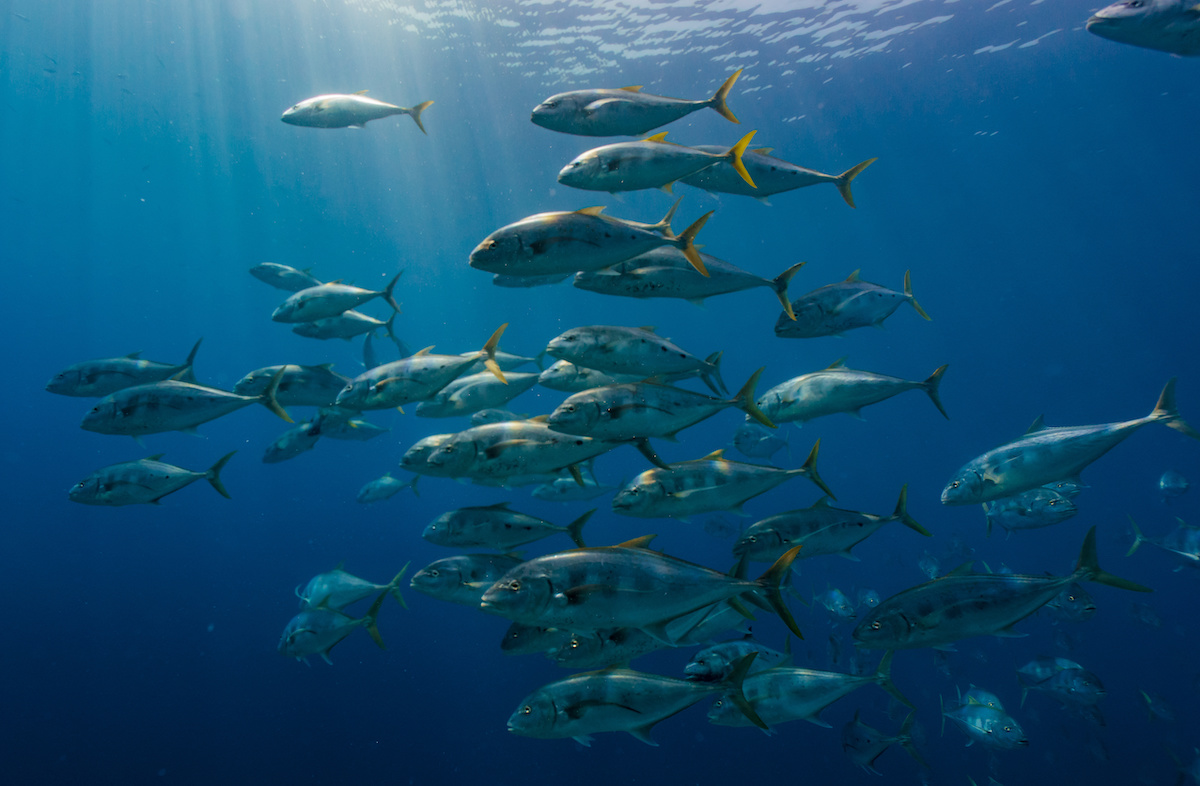In this underwater photograph, a school of approximately 20 to 30 medium-sized fish, likely bluefin tuna, swim gracefully towards the left side of the frame, revealing their full, streamlined profiles. Each fish displays a striking combination of silvery blue bodies adorned with distinctive yellow tails and fins, along with a hint of grayish striping along their sides. The scene is beautifully illuminated by sunbeams penetrating the surface of the water, casting gentle light patterns over the fish and highlighting their vibrant colors. The upper portion of the image showcases the ripple effects of the water's surface, while the background remains a serene, deepening blue, free of any other marine life or coral, emphasizing the purity and tranquility of this underwater moment.